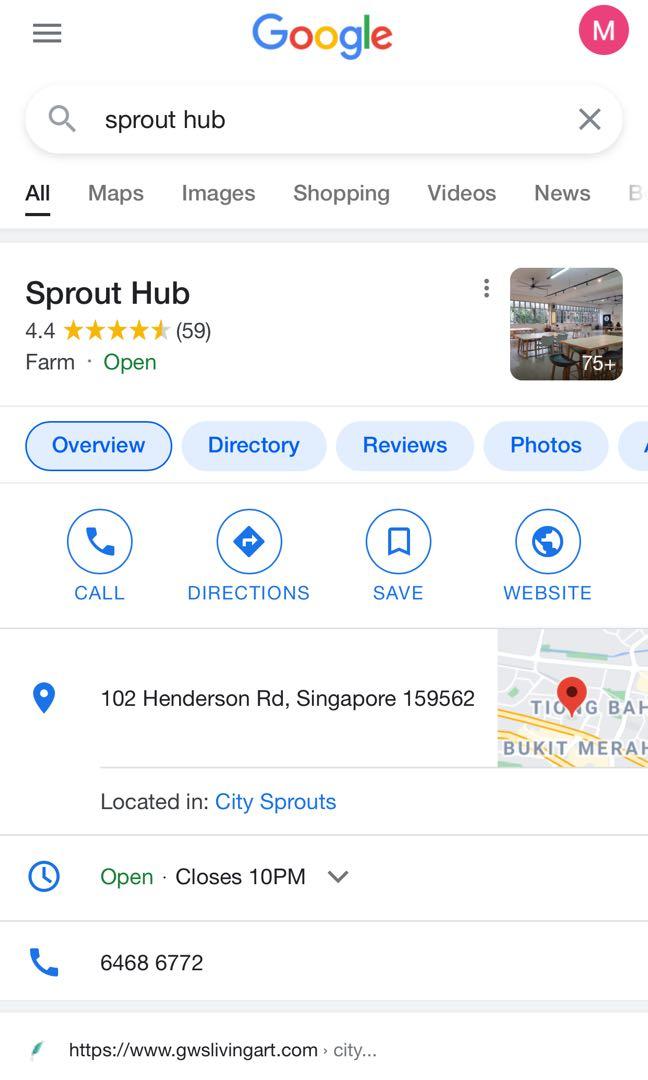The image is a screen capture of a Google search page displayed on a digital device. At the top center of the screen, the multi-colored Google logo is prominently featured in blue, red, yellow, blue, green, and red letters. Directly below the Google logo sits the search bar, which contains the phrase "sprout hub" written in black text. Underneath the search bar are the search display options, with the option "All" underlined, indicating it is currently selected. The search results for "sprout hub" are shown below the search display options. At the top of the results, "sprout hub" is displayed in large, bold, black text. Beneath this name, there is a rating of 4.4 stars, with the stars depicted in yellow. Adjacent to the stars is the number 59, signifying that the rating is based on 59 reviews. In the main body of the screen capture, additional details about Sprout Hub's location are also visible.